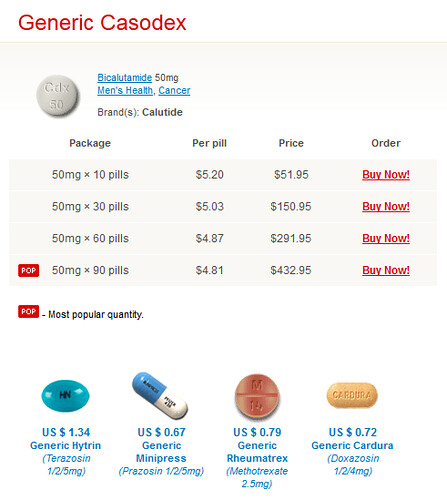This image is a detailed screenshot from a website where users can purchase prescription drugs online. The background is predominantly white. In the upper left corner, bold red text spells out "Generic Casodex." Directly below this, there is a subtle light gray border that is almost unnoticeable due to its faint hue.

Within the bordered section, an image of a gray pill is prominently displayed. The pill is imprinted with what appears to be the letters "CE" or "CDX," and just beneath the imprint, the number "50" is visible. To the right of the pill, "Bicalutamide" is written in blue font, followed by "50 mg" in gray font. Below this, the terms "Men's Health, Cancer" are underlined in blue, indicating a clickable hyperlink.

Further down, the word "Brand(s):" is written in gray, followed by "Calutide" in parentheses, emphasizing the brand name. 

The lower section of the screenshot features a table organized into four columns, providing options for different quantities of bicalutamide tablets. The quantities range from "50 mg x 10 pills" to "50 mg x 90 pills." The subsequent columns list the price per pill, the total price, and an "Order" column. Each row in the "Order" column has a red, underlined "Buy Now!" link for immediate purchase.

Beneath this table, there are images of four different pills, presenting additional product options. From left to right, these include:
1. A blue, oval-shaped pill.
2. A capsule with a blue top and a white bottom.
3. A pill in a brick-red color.
4. A gold-colored oval tablet.

Under each pill image, the prices and names are written in blue font, making it easy for users to identify and compare between different products.